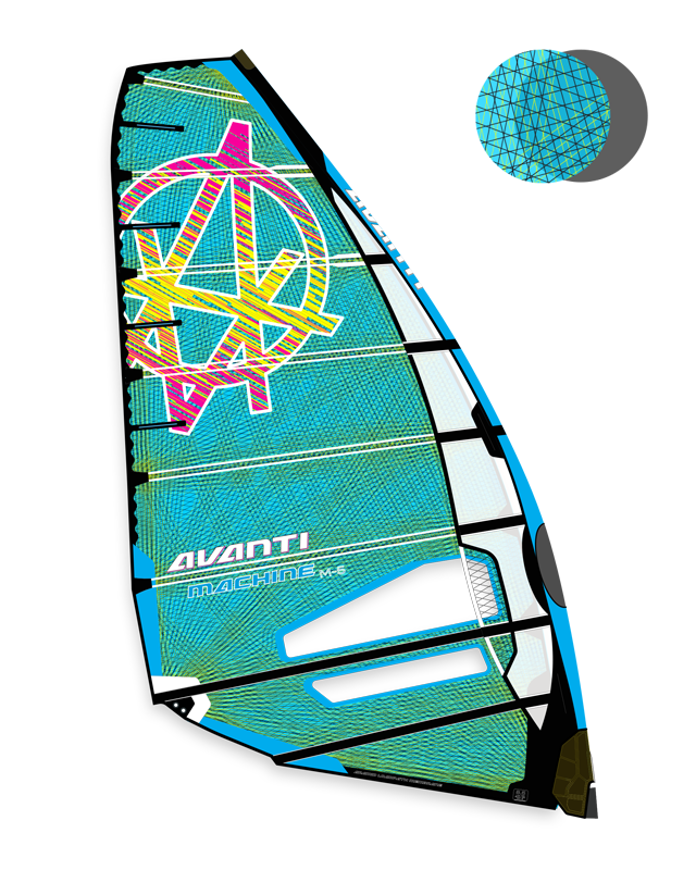The image shows a vibrant sail of a sailboat, which has a unique four-sided shape with the top side shorter and the right side longer and slightly curved outward at the center. The sail features a striking combination of primarily green and blue colors, accentuated by an elaborate geometric pattern of thin cross-hatched lines in light brown, black, blue, and green. This pattern creates a dynamic abstract design, adding to the sporty and eye-catching appearance of the sail.

In the upper part of the sail, there is a prominent circular emblem with a complex design that includes a pink, green, and yellow line pattern along its edge. Inside this circle, there are two "A" shapes, one inverted and one upright, contributing to the distinctive look of the sail. The center of the circle contains multicolored slashes, including bright yellow and blue, which contrast sharply against the green background of the sail.

The bottom left corner displays the brand name "Avanti" in large white letters, with the word "machine" written in blue beneath it. The outer edge of the sail is mostly black with some light blue sections, and there are dark black cross supports forming rectangular shapes across the interior. The sail appears to be lying flat against a plain white background, highlighting its intricate details and vibrant colors.